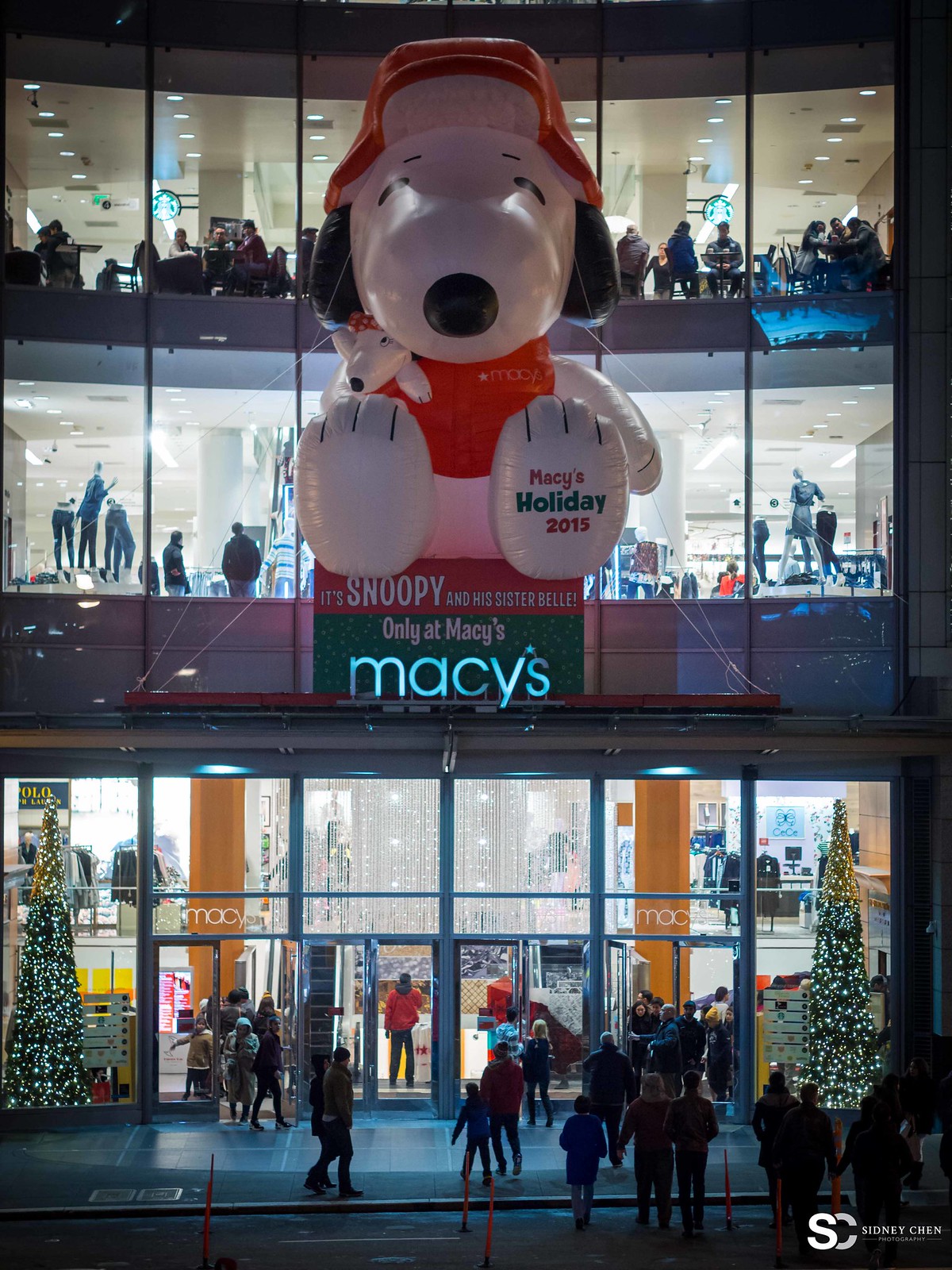This photograph captures the exterior of a three-story Macy's store during the Christmas season. The building features large transparent windows on each level, allowing the interior to be visible. The bottom level showcases bustling sidewalk activity with people entering and exiting the store. On either side of the entrance, slender, tall, and brightly lit Christmas trees adorn the doorway.

Inside, the first floor features people walking and shoppers browsing amongst mannequins in the clothing section, illuminated by bright lights and possibly an ornate glass chandelier. The second floor also displays shoppers and mannequins, while the top floor has a seating area where patrons can be seen sitting at tables.

Dominating the facade above the Macy's sign, which is prominently displayed in lit-up lowercase blue letters, is a giant inflatable Snoopy dressed in a red and white Santa hat and red sweater. Snoopy also holds a small doll and displays text on its right foot reading "Macy's IN RED, Holiday IN GREEN, and 2015 IN RED." This festive decoration, reminiscent of the Macy's Thanksgiving Day Parade balloons, highlights the store’s holiday theme. The photograph was taken at night, adding to the vibrant and festive atmosphere with the building and decorations well lit.